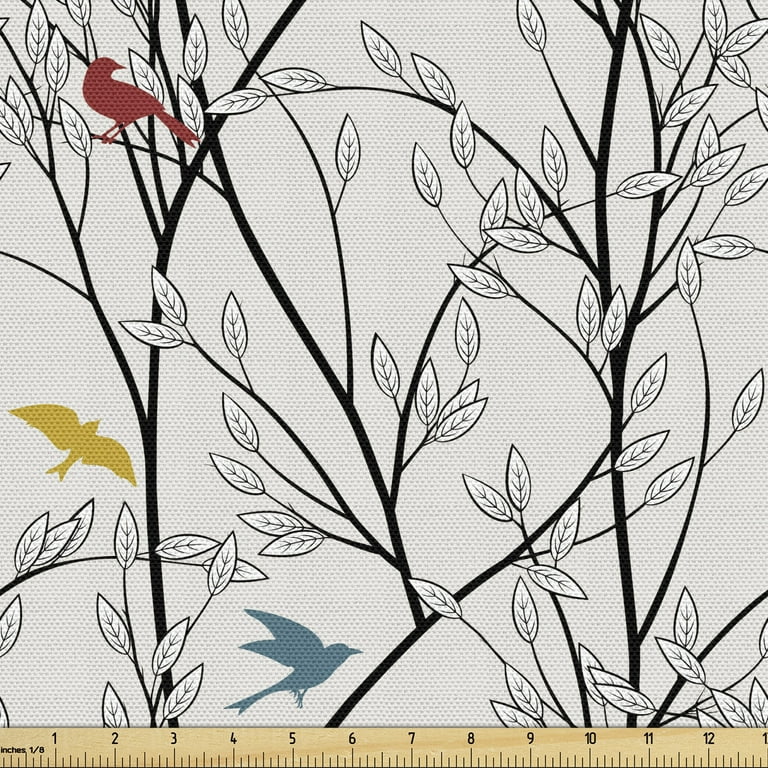Against an off-white, ivory background, the intricate drawing features a series of thin, black trees with delicate, sprawling branches adorned with numerous petite, white leaves, particularly dense towards the top part of the image. At the very bottom of the drawing runs a tan, hand-drawn ruler, marked in inches, extending up to 13, although the last number is slightly cut off. Among the trees, three colorful birds stand out vividly against the monochromatic scheme. In the upper left corner, a red bird perches gracefully on a branch, facing backward to the right. Below it, near the bottom left, a golden-yellow bird is captured mid-flight, ascending upwards. Further down, closer to the center-left, a blue bird, also in flight, heads towards the right. Each bird measures approximately two inches in length and height, adding a burst of color to the predominantly black and white scene.